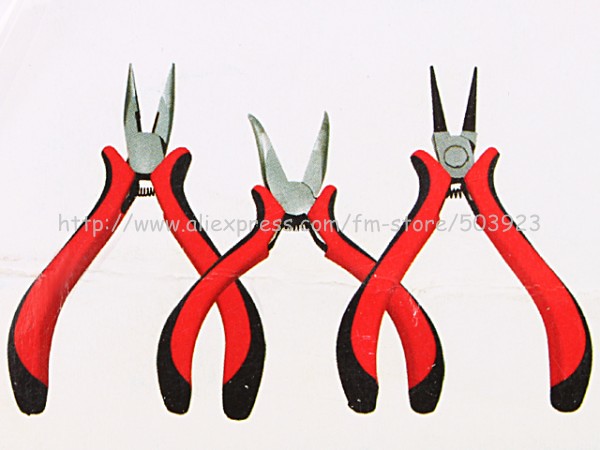This image is a detailed product photo of three pairs of pliers with red handles and black trim, arranged on a light green and pink background. Each pair of pliers features a different type of tip: the far-left pair has medium-length silver tips, the center pair has thicker silver tips, and the far-right pair has needle-nose black tips with visible black ridges just above the round section. The pliers on the right overlap slightly with the center pair, which in turn overlaps the left pair. There is also a watermark with the URL "http://www.aliexpress.com/fm-store/503923" centered in the image, indicative of an internet product listing. The pliers' handles are uniformly equipped with springs, and above a horizontal wrinkle in the background, the URL is also prominently displayed.